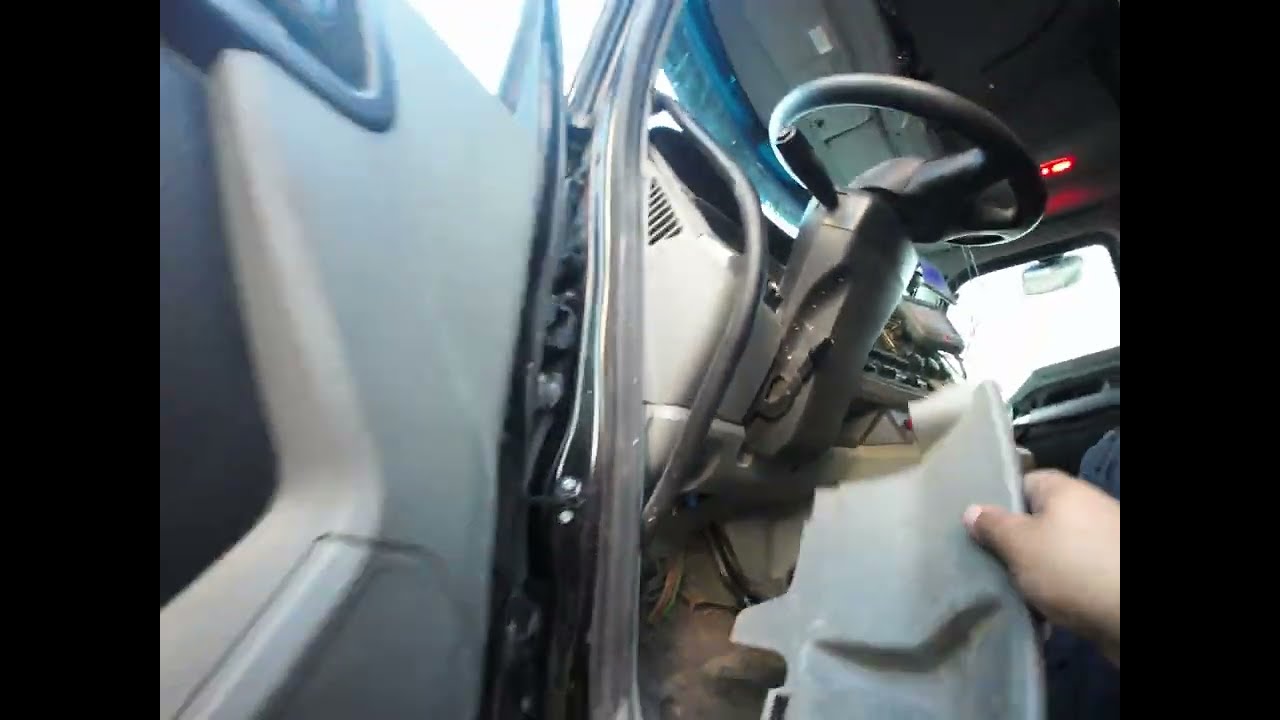Captured from a low angle just outside the vehicle, this image provides a detailed look inside a truck's cabin during daylight. The main focus is on the lower part of the dashboard beneath the black steering wheel, which appears dismantled. A right hand, positioned in the lower right corner of the image, firmly holds a torn fragment of gray plastic from the dashboard area. To the left, part of the driver's side door is visible, adding context to the setting. The photograph emphasizes the stark interior with a mix of colors, predominantly gray, off-white, red, blue, white, and brown. The overall impression suggests a worn and heavily used vehicle interior.